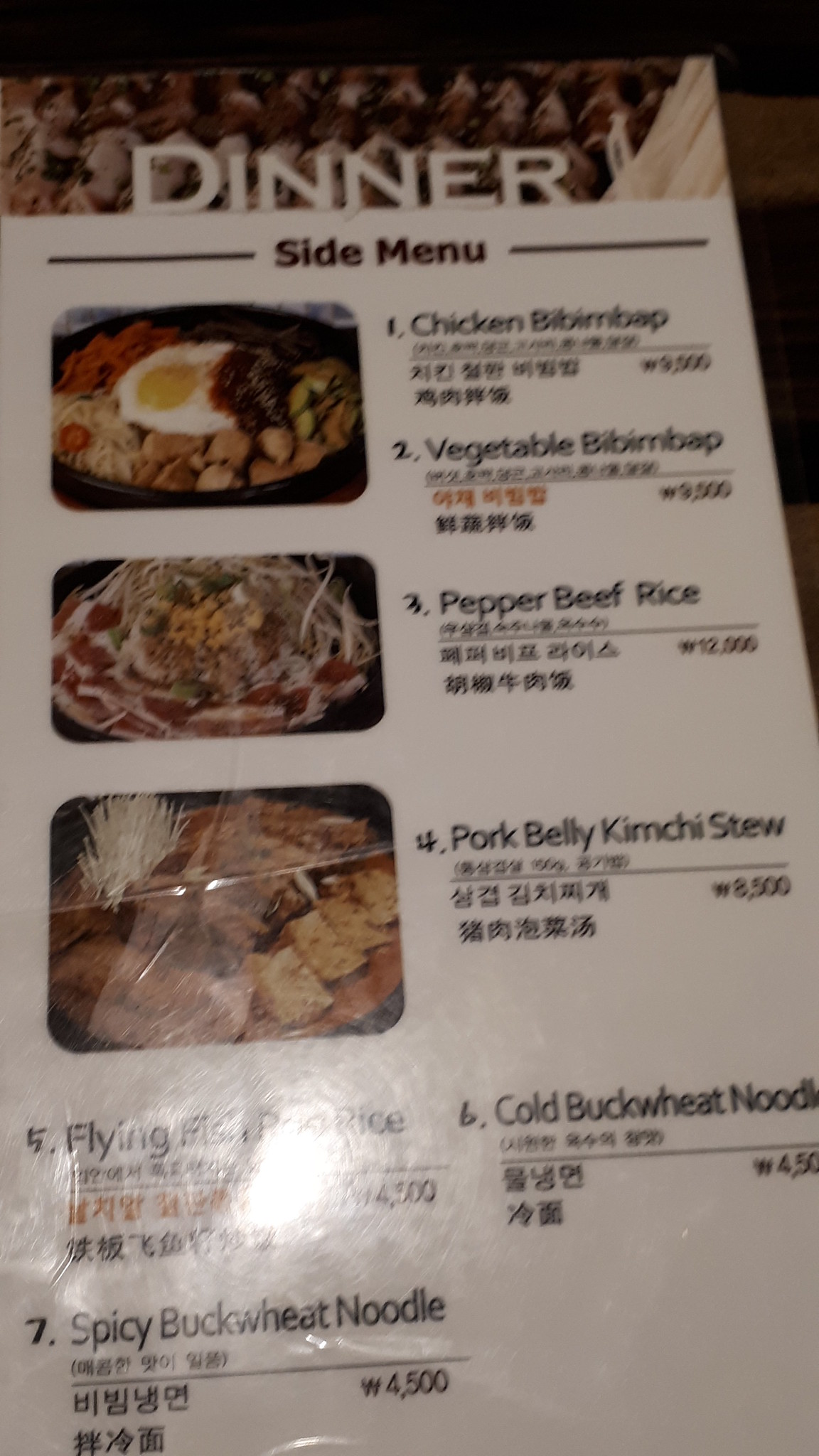A close-up image of a laminated menu, showing a section titled "Dinner" in white letters at the top, with "Side Menu" written below in darker letters. Straight lines border the menu edges for visual detail. The first item listed is "Chicken Bibimbap," accompanied by a small image of the dish. Beneath the English title, there are Asian characters and an obscured price. The second item is "Vegetable Bibimbap," similarly featuring a dish image, Asian characters, and an obscured price. The third item, "Pepper Beef Rice," follows the same format. The fourth item is "Pork Belly Kimchi Stew," with its description and price in Asian characters below, and the dish image. The bottom section lists three additional items without photographs. The fifth item is partially obscured by a glare, with only the word “Flying” visible. The sixth item, "Cold Buckwheat Noodles," includes a description and price. The seventh item, "Spicy Buckwheat Noodles," is listed in the same format.